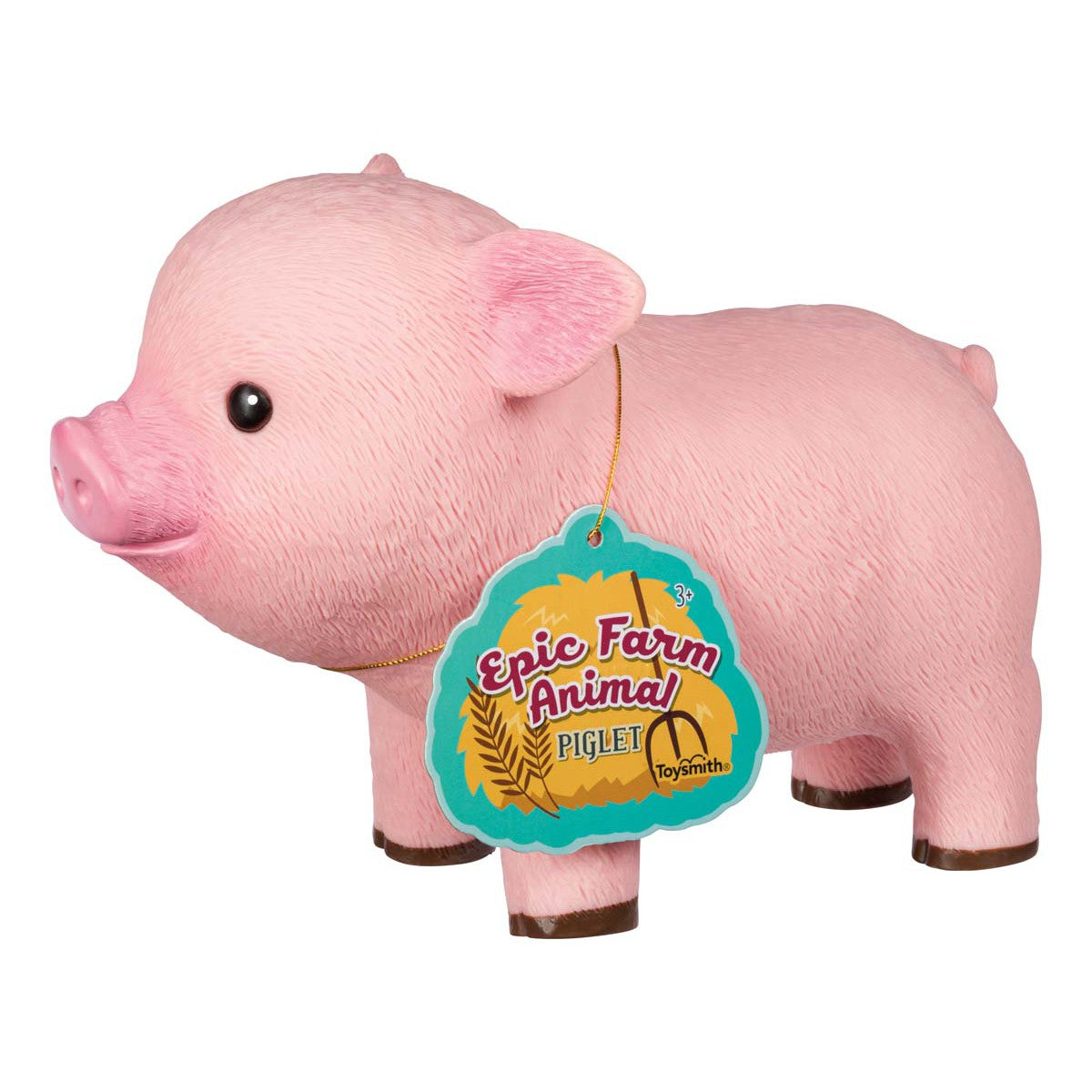The image depicts a pink toy piglet facing left, made of plastic or resin, giving it a slightly 3D illustrated look. The piglet features a brighter pink nose and ear insides, a light pink body, dark brown hooves, and a single beady black eye with a white dot. It has a gold string around its neck attached to a teal tag with a lighter teal outline. The tag showcases a tan haystack with a pitchfork and wheat on the left, set against a white background. The text "Epic Farm Animal" is displayed in dark red, bubbly cursive font, outlined in white, followed by "Piglet" in black normal lettering, also outlined in white. At the bottom right of the tag, "Toysmith" is printed in black lettering.